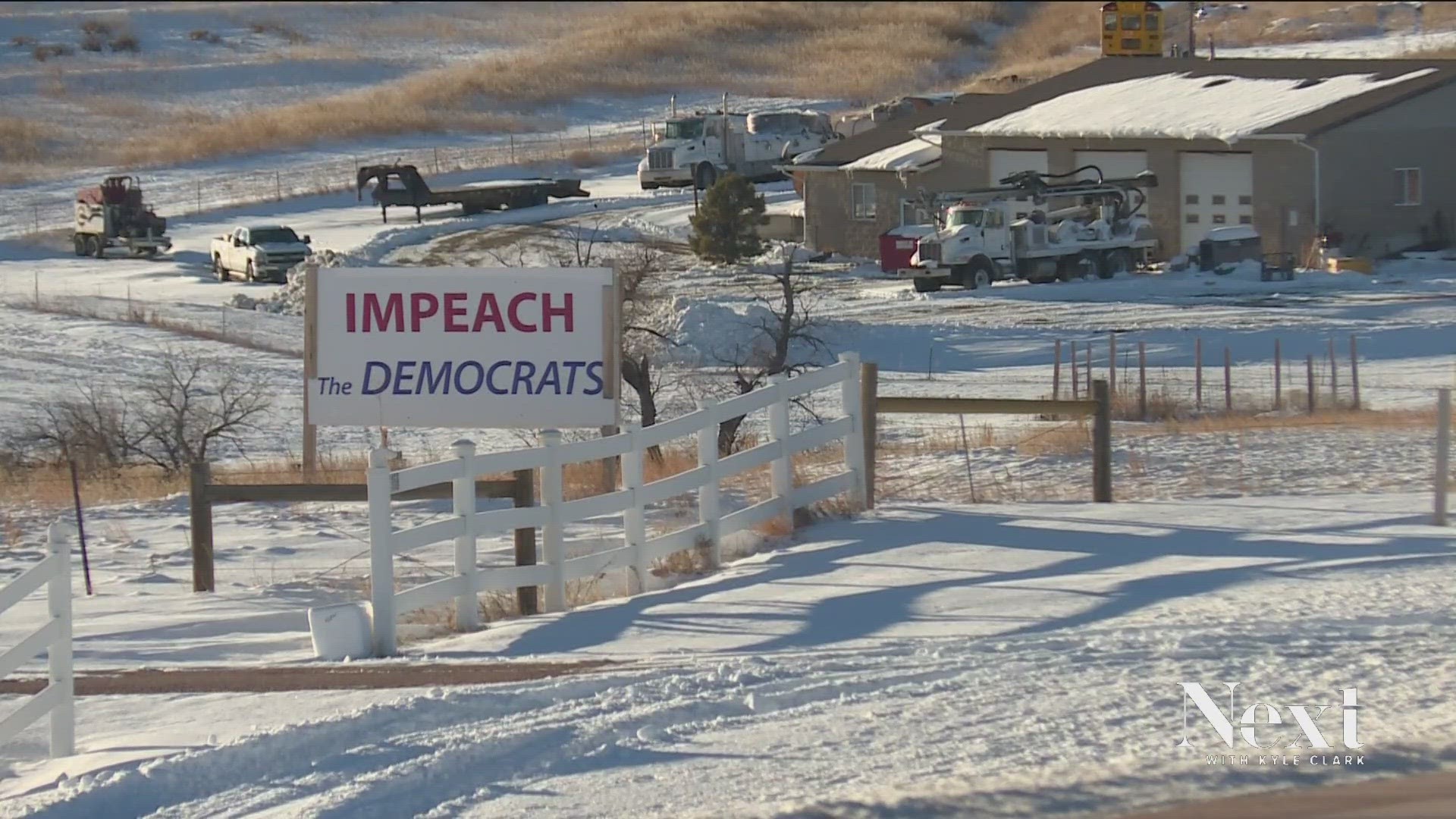This photograph, possibly taken for news reporting, showcases an outdoor snowy scene, likely captured in a remote, possibly Western, rural area. A large white sign with bold red letters reading “Impeach” and blue letters stating “the Democrats” stands prominently on two wooden pillars, making it the focal point of the image. The sign is positioned in front of a white, gated wooden farm fence, with a white cooler sitting nearby.

In the background, there is a building, likely a repair shop or manufacturing facility, featuring three large garage bays. Numerous specialized work vehicles, including a large white truck with specialized equipment, a pickup truck, an 18-wheeler, and other trucks and tractor-trailers, are parked around the property. The snowy ground contrasts with patches of dry, dead grass and leafless trees, indicating a late winter season.

The scene captures long shadows, suggesting a sunny day despite the snow. In the lower right corner, the text "Nexi" followed by "Kyle Clark" can be seen, possibly indicating the photographer or the source of the photo. The landscape around the area includes hills covered with yellowish brush, further emphasizing the rural and remote setting.